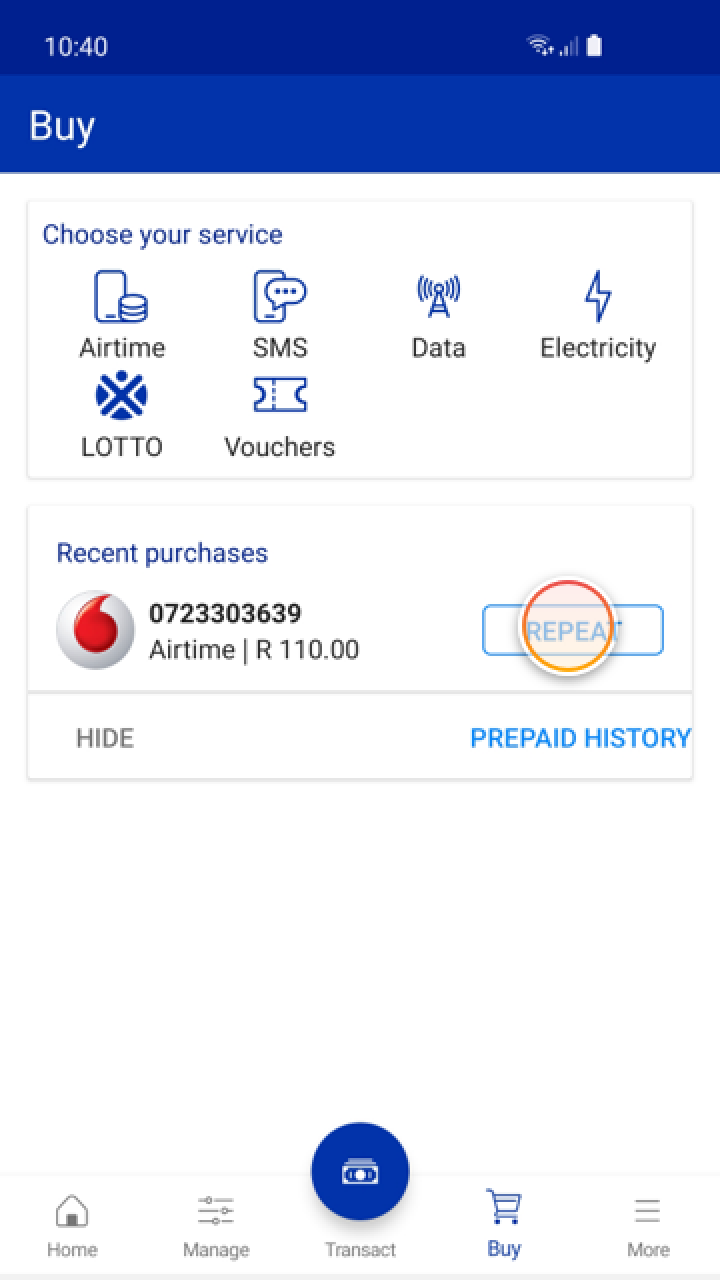The image depicts a standard bank app displayed on a smartphone. The top section of the app, colored blue, features the word "BUY" on the upper left corner. Below this header, the page presents the section labeled "Choose Your Service" in blue text, with various service options illustrated in blue and text written in black. The service options available are: A-Time, SMS, Data, Electricity, Lottery, and Vouchers.

Further down, the app displays a section titled "Recent Purchases," which records an A-Time purchase amounting to 110 Rands. The associated phone number for this transaction is 0723303639. Located to the left of the phone number is the Vodacom logo, indicating that the A-Time purchased was for a Vodacom service. The logo is circular, featuring a white exterior and a red interior. On the right side of the recent purchase information, there is a blue "REPEAT" button, accentuated by an orange circle with a white outline pointing towards it.

Below this section, on the bottom right, it says "Prepaid History" in blue text, while on the bottom left, it says "Hide" in grey text. At the very bottom of the app, there are five navigation buttons. From left to right, they are: Home, Manage, More, Buy (which is highlighted in blue), and a central button, presumably for transactions, marked by a blue and white intersecting line design.